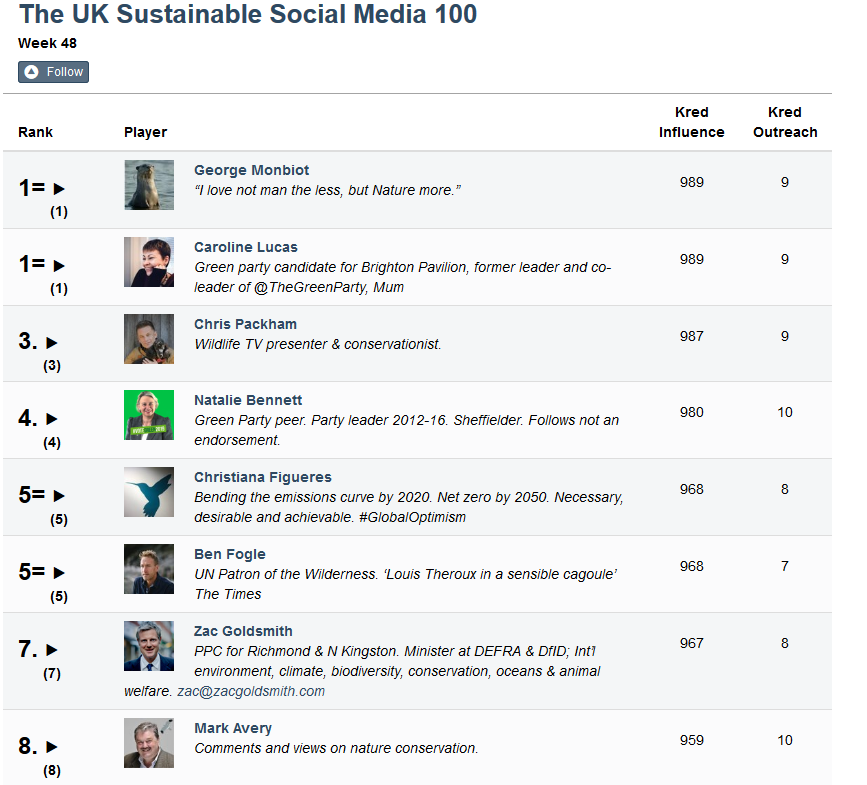In the top left corner of the image, the title "UK Sustainable Social Media 100" is prominently displayed in blue, followed by "Week 48" in black. The word "Follow" is also visible, enticing viewers to engage with the content. 

The main part of the image features a ranked list of influential social media personalities in the UK sustainability sector. The "Rank" column on the left has various numbers indicating their positions: the top two entries have "1=", both pointing to the right with a blue arrow, denoting a tie. Subsequent ranks are listed as 3, 4, and then two entries tied at 5 and labeled "5=", followed by 7 and 8.

Next to the rank column, the "Player" column lists the influential individuals along with small images and brief descriptions:
1. **George Monbiot** - Below his name, a quote is displayed: "I love not man the less but nature more."
2. **Caroline Lucas** - Identified as the Green Party candidate for Brighton Pavilion and former leader and co-leader of the Green Party.
3. **Chris Packham**
4. **Natalie Bennett**
5. **Christiana Figueres**
6. **Ben Fogle**
7. **Zac Goldsmith**
8. **Mark Avery**

The final columns, "Cred Influence" and "Cred Outreach," contain numerical values reflecting their social media influence and reach. The "Cred Influence" scores for these individuals are mostly in the 900s, while "Cred Outreach" ranges from 7 to 10, indicating their impact and engagement on social media platforms.